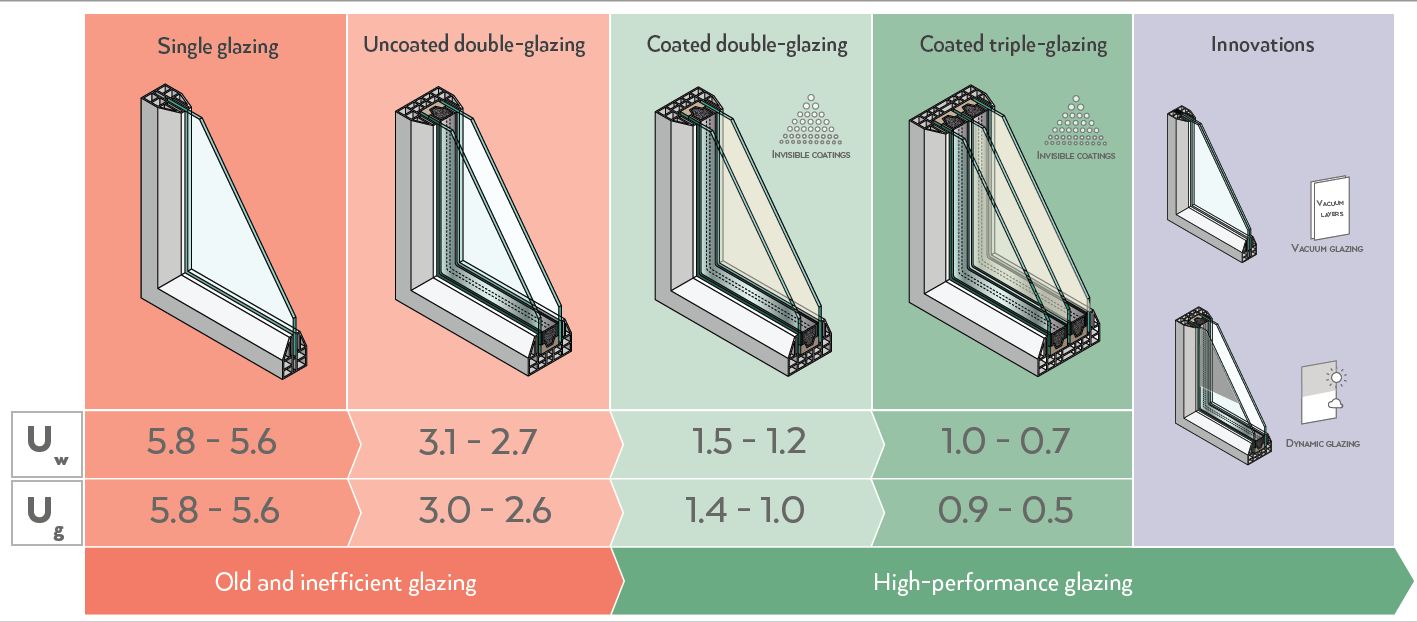The illustrated chart details the different types of window glazing, highlighting their performance levels and innovations. The topmost section, labeled in dark gray, categorizes the glazing types into single glazing, uncoated double glazing, coated double glazing, coated triple glazing, and innovations. Each category is represented with a cross-sectional diagram of a window pane, showing one pane for single glazing, two panes for uncoated double glazing, coated double glazing, and three panes for coated triple glazing. The innovations section includes two images depicting advanced glazing techniques with a single pane and a double pane. Beneath each image, detailed numerical values for UW and UG performances are provided, showcasing a progressive improvement from inefficient to high-performance glazing: single glazing (5.8 to 5.6), uncoated double glazing (3.1 to 2.7), coated double glazing (1.5 to 1.2), and coated triple glazing (1.0 to 0.7). The chart uses a color gradient to signify glazing efficiency, starting with a peachy hue for old and inefficient types (single and uncoated double glazing) and transitioning to green for high-performance glazing (coated double and triple glazing), culminating in the gray-labeled innovations category, representing the latest advancements in window technology.